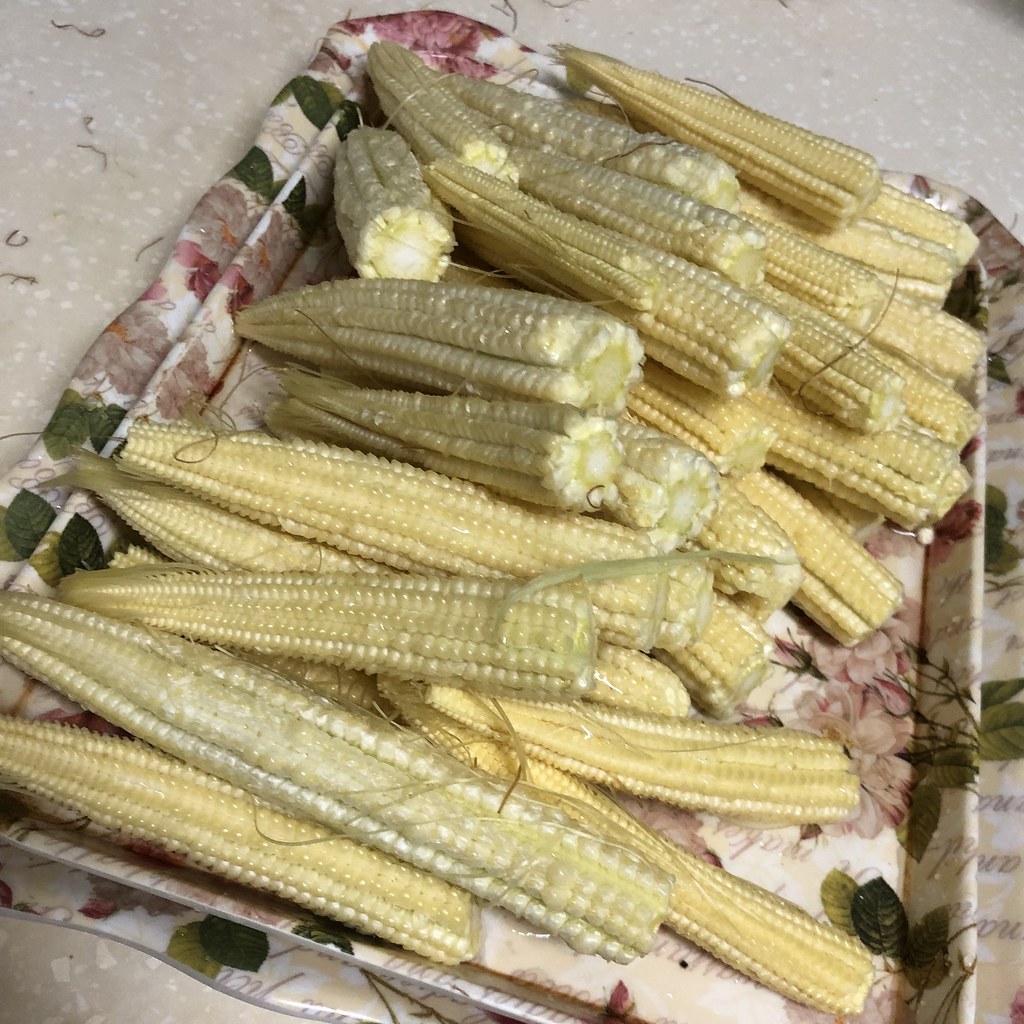A delicate, rectangular platter adorned with a floral print featuring shades of pink and green leaves sits atop a beige countertop. On this ornate tray, which is scalloped and about two inches deep, lies a bountiful pile of thin, miniature ears of corn. Approximately 40 to 50 ears, varying in shades from bright yellow to a slightly grayish tint, are haphazardly stacked, showcasing a mix of underdeveloped kernels and remnant silk fibers from the shucking process. Some of the corn still clings to small green leaves and brown tassels. The platter's intricate floral design, combined with its vibrant yet modest corn offering, creates a striking contrast against the plain, dotted white table backdrop.